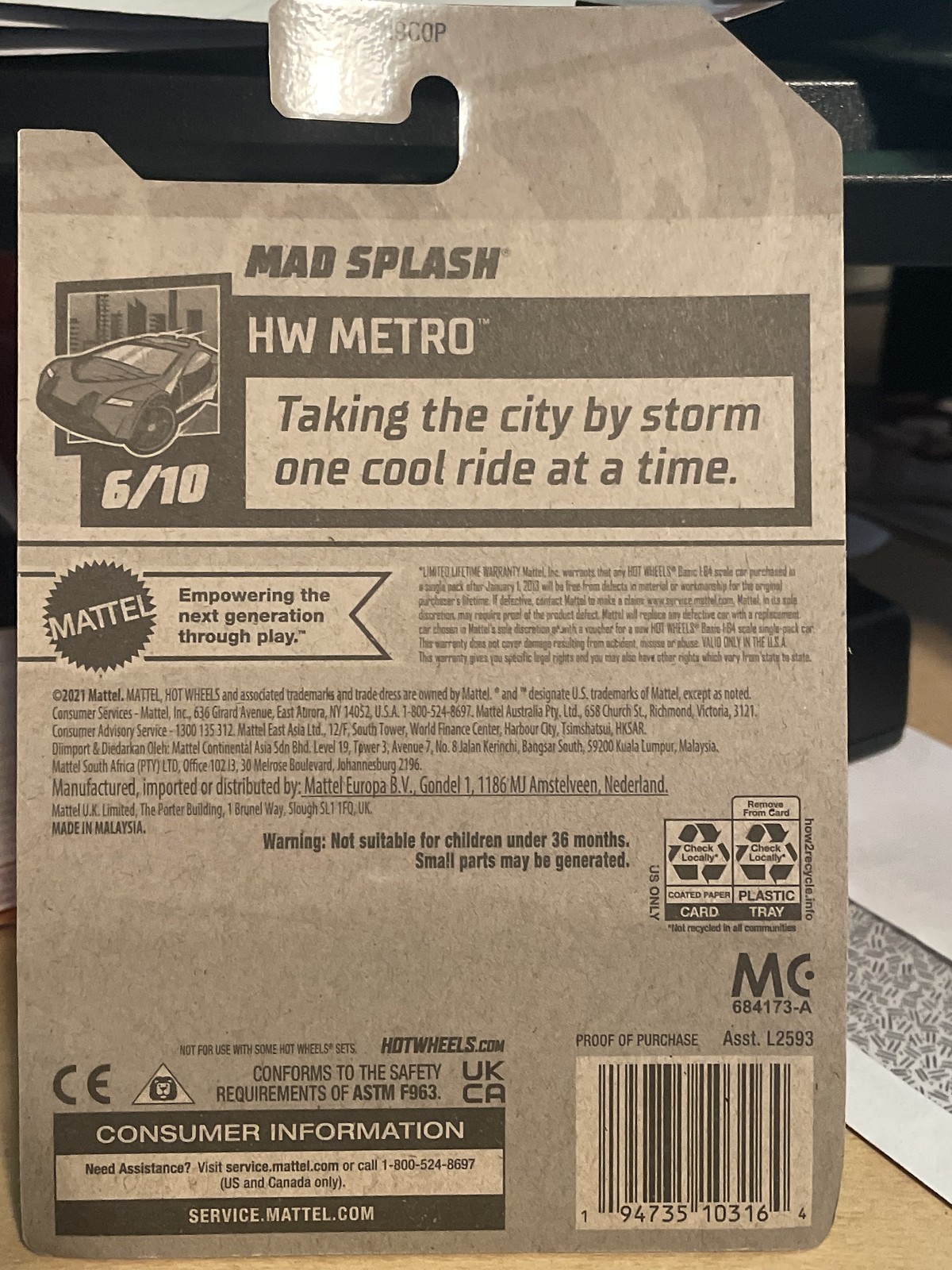The image depicts the back cover of a Hot Wheels product. Dominating the top portion is the bold title "Mad Splash." Just below, within a black rectangular box, the text reads: "HW Metro - Taking the city by storm one cool ride at a time." Adjacent to this, there is an illustration of a car accompanied by the numbers "6/10" beneath it. Positioned in the middle left section of the image is the iconic Mattel logo, paired with the slogan, "Empowering the Next Generation Through Play." To the right and extending below this area, various pieces of legal information are displayed, including copyright details and the manufacturing address, amongst other legal disclaimers.